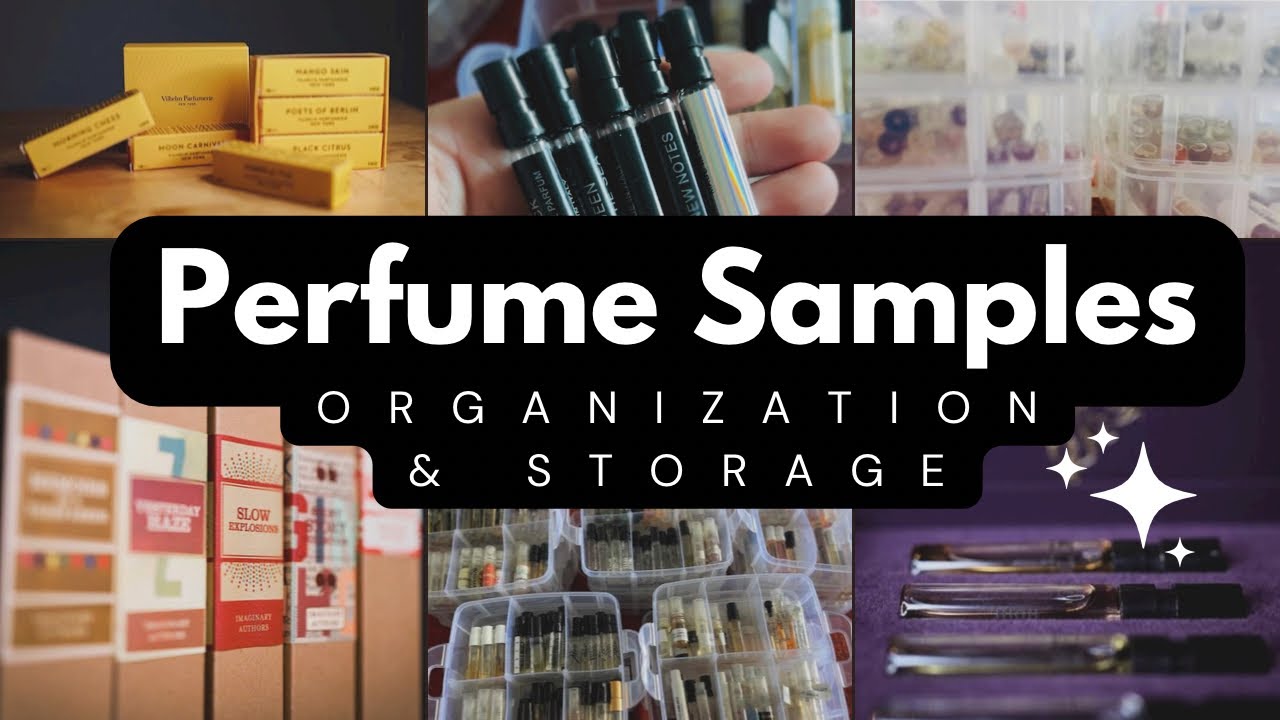The image is a collage composed of six smaller photographs arranged in a rectangular layout, with three pictures on the top row and three on the bottom row. At the center of this rectangular formation, there is a black area with white text that reads "Perfume Samples, Organization, and Storage." The corners of the black area are rounded, adding a soft touch to the design. Below the text, four stars are drawn in the bottom right corner - one larger star with three smaller stars accompanying it.

The images depict various methods of organizing and storing perfume samples. At the top left, there are some yellow boxes with labels, positioned on a wooden surface. In the top middle, a hand holds five glass vials with black plastic caps, each containing different colored liquids. The top right image shows some clear plastic containers, albeit blurry, suggesting they hold additional storage items.

On the bottom left, you see labeled cardboard boxes. The bottom middle image displays more plastic storage cases, meticulously organized with perfume vials inside. Lastly, the bottom right photo features a collection of perfume vials arranged in a purple, velvety container, with the vials neatly inset within the fabric to keep them in place. Together, these images provide a comprehensive overview of different storage solutions for perfume samples.